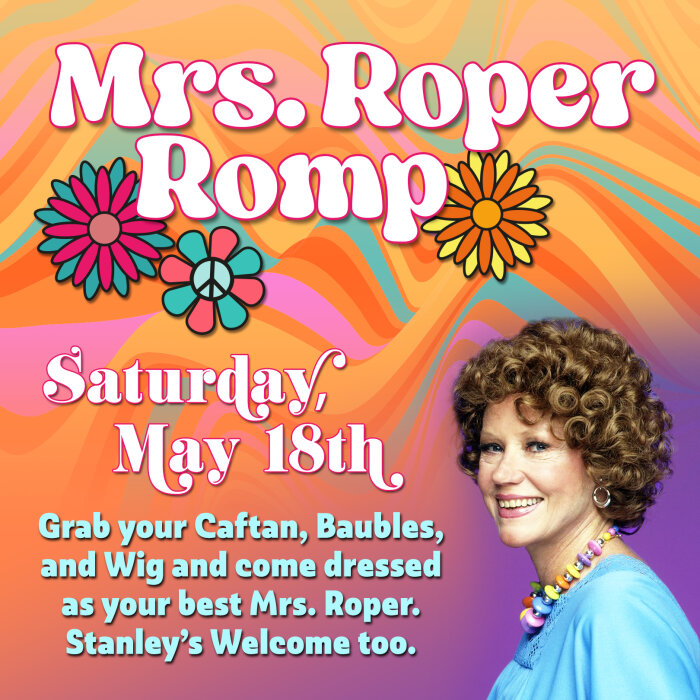The flyer is a vividly colored advertisement for the "Mrs. Roper Romp" event, featuring a psychedelic background in orange, blue, pink, yellow, and purple waves. The title "Mrs. Roper Romp" is adorned with three large flowers; a yellow and orange one on the right and blue and pink ones on the left, one of which contains a peace sign. Below the flowers, the event date, "Saturday, May 18th," is prominently displayed. The bottom left corner invites attendees with the message: "Grab your caftan, baubles, and wig, and come dressed as your best Mrs. Roper. Stanleys welcome too." The right-hand side showcases a picture of a woman with short, curly brown hair, smiling while wearing a blue dress and a necklace with large, brightly colored beads in pink, purple, yellow, orange, and blue. The overall design evokes a lively and nostalgic feel, reminiscent of the fun and iconic style of Mrs. Roper.